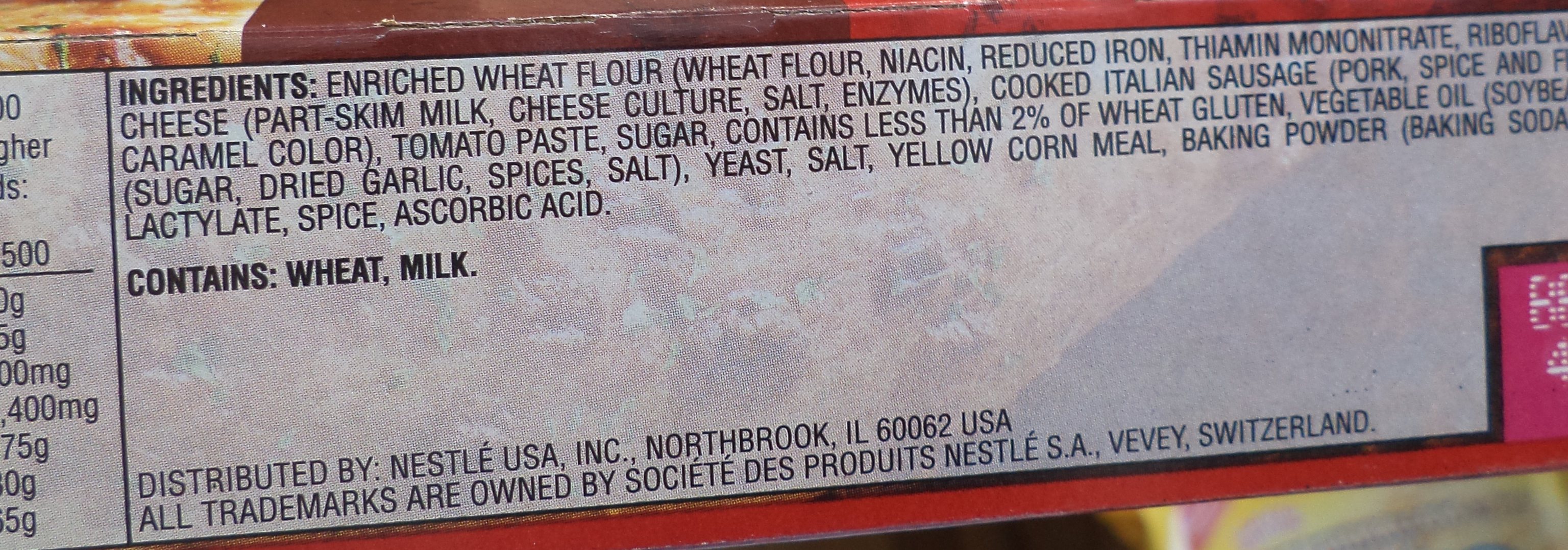The image features a close-up of a narrow, horizontal, rectangular product label on the back of a red carton, most likely a Nestlé product. The white label, framed by a red border, lists various ingredients in black text. The main ingredients include enriched wheat flour (with nutrients like niacin, reduced iron, thiamine mononitrate, and riboflavin), part-skim milk cheese (cheese culture, salt, and enzymes), cooked Italian sausage (pork, spices, and flavorings), caramel color, tomato paste, and sugar. It also mentions that the product contains less than 2% of wheat gluten, vegetable oil (soybean), dried garlic, spices, salt, yeast, yellow cornmeal, baking powder (baking soda), lactylate, spice, and ascorbic acid. The label explicitly states it contains wheat and milk. At the bottom, it notes that the product is distributed by Nestlé USA, Inc. in Northbrook, Illinois, and all trademarks are owned by Societies des Produits Nestlé S.A., Vevey, Switzerland. The background includes bits of white, yellow, and pink colors at the lower right-hand corner, as well as a mix of tan and dark brown hues at the upper left, providing additional context to the package’s design.